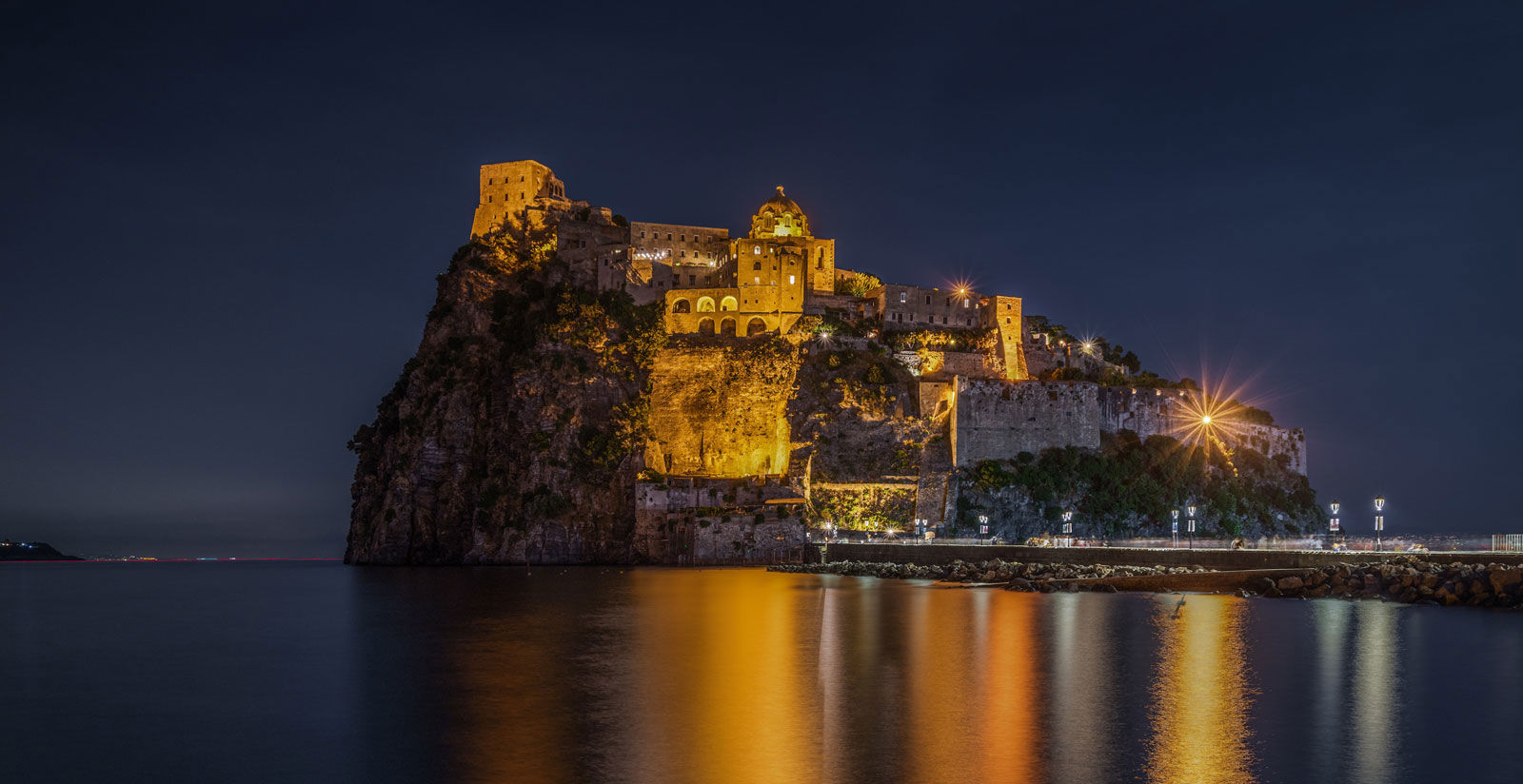This horizontally rectangular, full-color photograph showcases a striking nocturnal scene of an island resembling a fortress or castle, situated in calm water. The island is adorned with a collection of illuminated buildings that exude a warm, golden glow, reminiscent of a religious site like a cathedral. A lengthy, well-lit walkway extends from the lower right corner of the image, connecting the island to either a bridge or an adjacent landmass. This path features visible signs or lampposts along its length. The night sky above is a deep, almost cloudy dark blue, devoid of stars, but with distant city lights possibly visible in the far background. The tranquil water surrounding the island mirrors the picturesque lighting, adding to the serene and majestic atmosphere of the scene, which is seemingly viewed from another piece of land or possibly a boat.